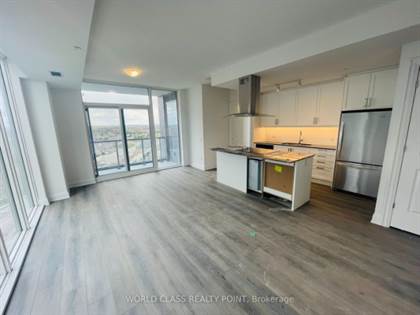This is a detailed architectural rendering of a compact high-rise apartment, prominently showcasing the kitchen area situated on the left side. The kitchen features a sleek, modern design with a small island serving as both a workspace and a potential dining area. Behind the island, there is a minimalist sink setup accompanied by a large, stainless steel refrigerator, contributing to the contemporary aesthetic.

The room is bathed in natural light from tall, expansive windows that line the walls, offering a panoramic view and creating an open, airy ambiance despite the apartment's limited square footage. The flooring throughout the space is composed of light-colored wood, enhancing the bright and welcoming atmosphere.

At the bottom of the image, a nearly transparent overlay reads "World-Class Realty Point Brokerage," indicating that this sophisticated and efficiently designed space is available for lease or purchase through a real estate website. The photo has been meticulously edited, with all borders removed to present an uninterrupted view of the area. Notably, the space is unfurnished, allowing potential tenants or buyers to envision customizing it to their individual tastes.